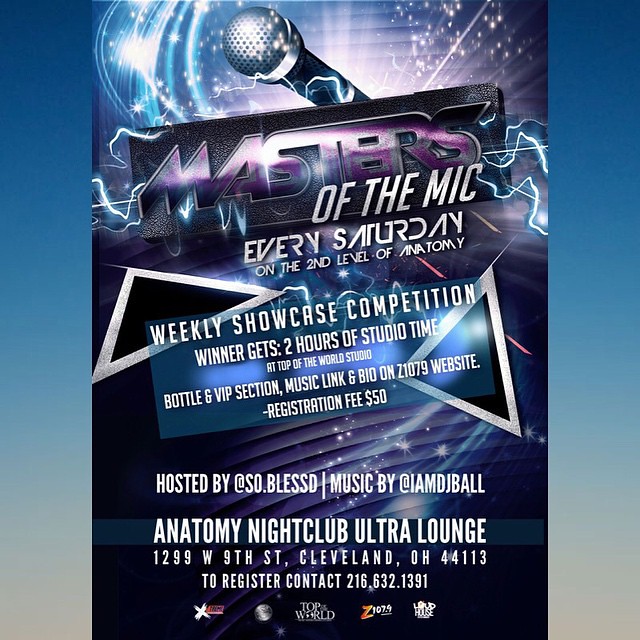The image predominantly features a vibrant poster for a weekly social competition called "Masters of the Mic," held every Saturday on the second level of Anatomy nightclub and ultra lounge. The centerpiece of the poster showcases a microphone with a silver head and a black handle against a sparkly blue and white background, with fireworks, stars, and spotlights adding a celebratory flair. The text "Masters of the Mic" is prominently displayed in purplish letters with lightning bolts, highlighting the excitement of the event. 

Underneath, it details that winners will receive two hours of free studio time at Top of the World Studio, a bottle, and a VIP session. Additional competition information and registration, which requires a $50 fee, can be found by following a music link and bio on the Z1070 website. The event is hosted by www.selfrested.com, with music provided by www.IamDJBo. The poster's edges have vertical blue lines, transitioning to a lighter gray at the bottom, adding to its dynamic and eye-catching design.